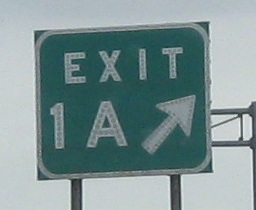The photograph captures an outdoor scene featuring a prominent interstate exit sign, which dominates the composition. The sign is a vibrant green with a crisp white border, extending to the corners which are also green rather than rounded. This detail gives the sign a distinctive appearance. Clearly printed in white, the sign displays "Exit 1A" alongside a diagonal arrow pointing upwards to the right, indicating the direction of the exit. The sign is securely mounted on a sturdy bar that spans its width, with two additional bars running vertically down to the ground for extra support. To the right, there are two poles seemingly connected to the sign, adding to its stable configuration. The overall image provides a detailed look at the functional and structural elements of wayfinding signage on highways.